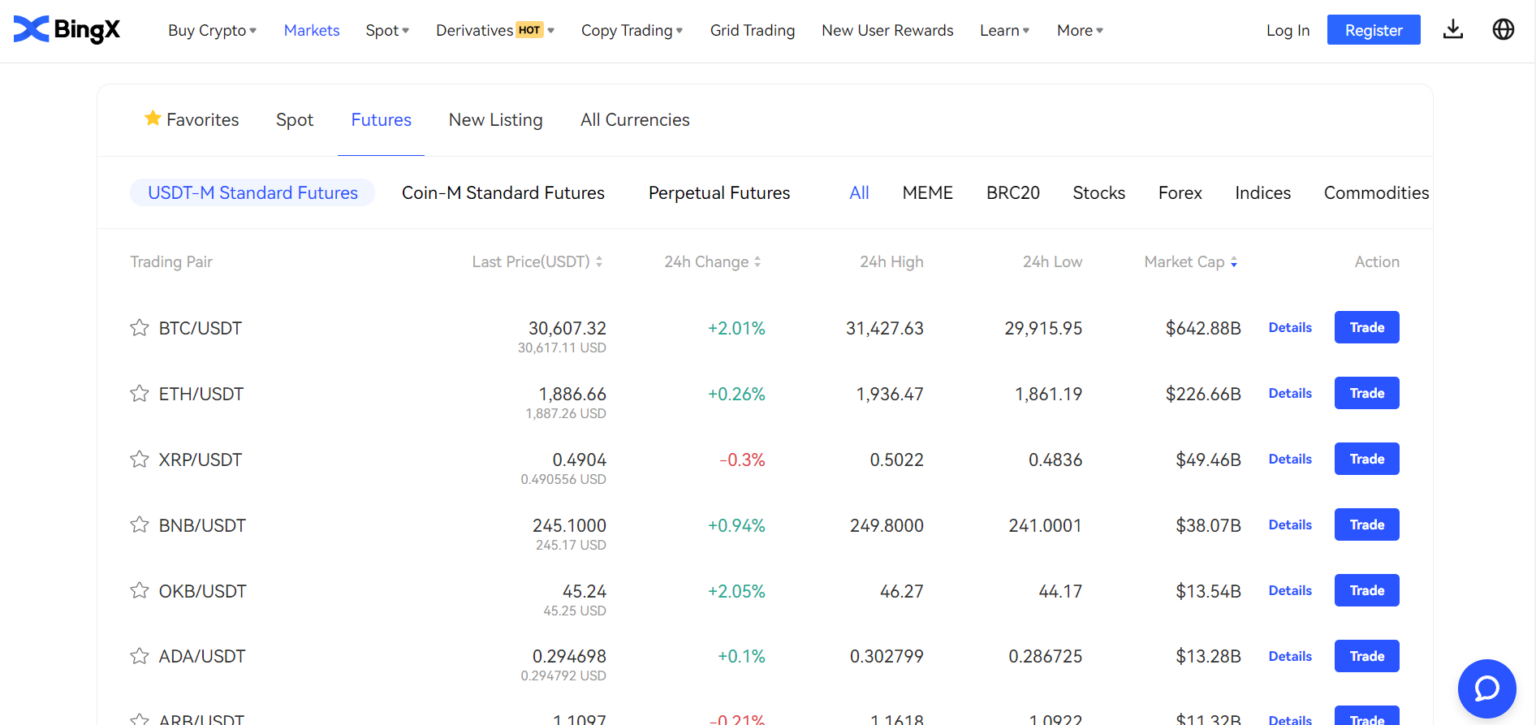The image features a clean interface of a cryptocurrency trading platform. At the top, there's a prominent blue "X" icon associated with BingX, alongside various sections such as "Buy Crypto," "Markets," "Spot," "Derivatives," "Copy Trading," "Grid Trading," "New User Rewards," "Learn," and a "More" option. To the right of these sections, there is a "Login" button next to a "Register" button, followed by a "Download" button. Adjacent to these, a globe icon is visible, indicating language or regional settings.

Beneath these icons, a series of tabs can be seen, labeled "Favorites," "Futures," "New Listing," and "All Currencies." The subsections under these tabs include "USDT-M Standard Futures," "Coin-M Standard Futures," and "Perpetual Futures." Further categories are listed below, including "All," "MeMe," "BRC 20," "Stocks," "Forex," "Indices," and "Commodities."

The main trading interface displays columns with headings: "Trading Pair," "Last Price (USDT)," "24 Hour Change," "24 Hour High," "24 Hour Low," "Market Cap," and "Action," providing detailed information on various trading pairs and their market metrics.

This image comprehensively illustrates a well-structured and feature-rich cryptocurrency trading dashboard designed to cater to both new and experienced users.